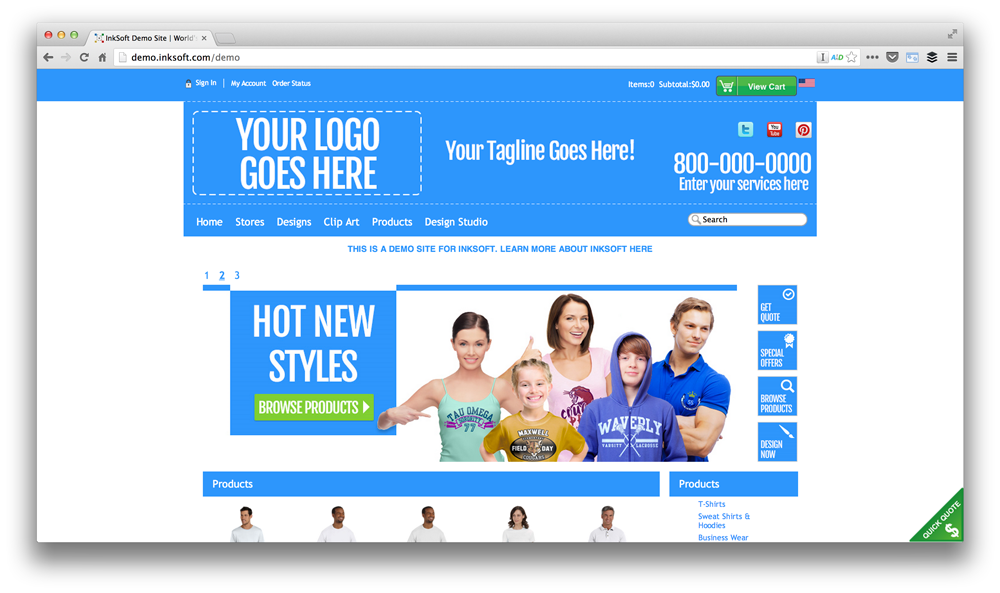The image depicts a webpage from the URL demo.inksoft.com/demo. At the top of the webpage, a blue horizontal line stretches across the width. Below this line, a blue section prominently displays the text, "Your logo goes here," in white letters, followed by "Your tagline goes here" in white lettering next to it. An 800 number is also listed in white within this section. The navigation menu includes options such as Home, Stores, Designs, Clip Art, Products, and Design Studio, accompanied by a search bar.

The background of the webpage is predominantly white. Directly underneath the navigation menu, there is a section titled "Hot New Styles" featuring an image of a smiling family, which appears to consist of a mom, dad, and three children. This section includes a button labeled "Browse Products" to explore the available offerings, which are highlighted under the header "Hot New Styles." 

Adjacent to the family image, there are four light blue boxes, adding to the structured layout of the page. At the bottom of the webpage, there is a blue bar labeled "Products," and a separate, disconnected blue bar below that with the same label. Below these bars, additional images are displayed in white, although these images are partially cut off in the view provided.